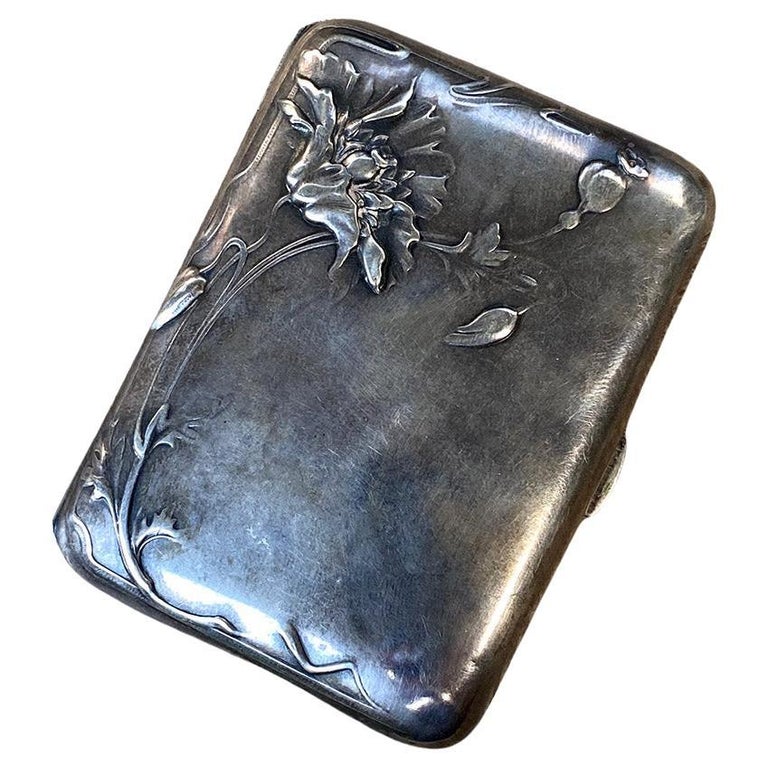The image depicts a polished silver metal case, akin to a nearly square cigarette holder with rounded edges, slightly tilting to the right and balanced on one corner. The case is adorned with intricate etchings, primarily featuring a floral design. A central flower with beautifully rounded petals grouped tightly in the center, colored in silver with mixes of black, highlights the top left corner. The flower’s stem extends from the bottom left, traverses the bottom in a zigzag pattern like a snake, and sprouts another flower towards the top right, finishing in swirling lines. There are also other elements, including a teardrop-shaped petal or bulb and a round spot at the top. The dark gray case has white scratches scattered across its surface and is set against a white background. Notably, there is a small lever or clasp positioned on the right edge for opening the case.